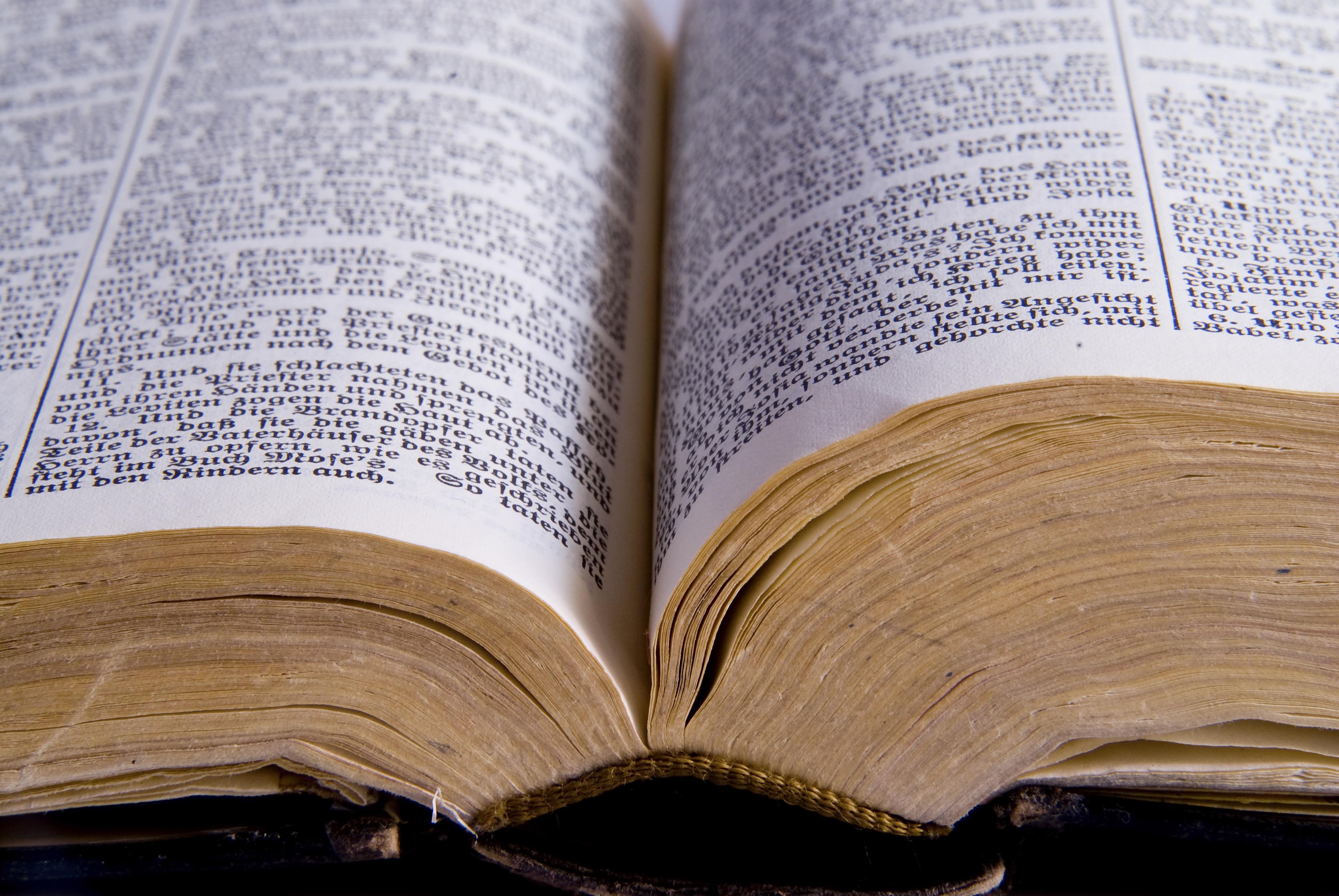This close-up image captures an old, thick, leather-bound book, likely a German-language Bible from approximately a century ago. The book is open and lying on a table, showing its spine and the divide between its pages, which are centered perfectly within the shot. The text is printed in an old-style German font, featuring numbered verses, suggesting it is a Bible. The open pages are brightly illuminated by a white light, revealing two columns on each page, for a total of four columns across the visible spread. The edges of the pages exhibit a yellowish to brown tint, indicative of aging, while the center, or “valley” between the pages, descends into a darker yellow hue. The binding, resembling a tweed cord of yellowish-brown color, along with the yellowing ends of the pages, adds to the vintage and heirloom quality suggested by the image.